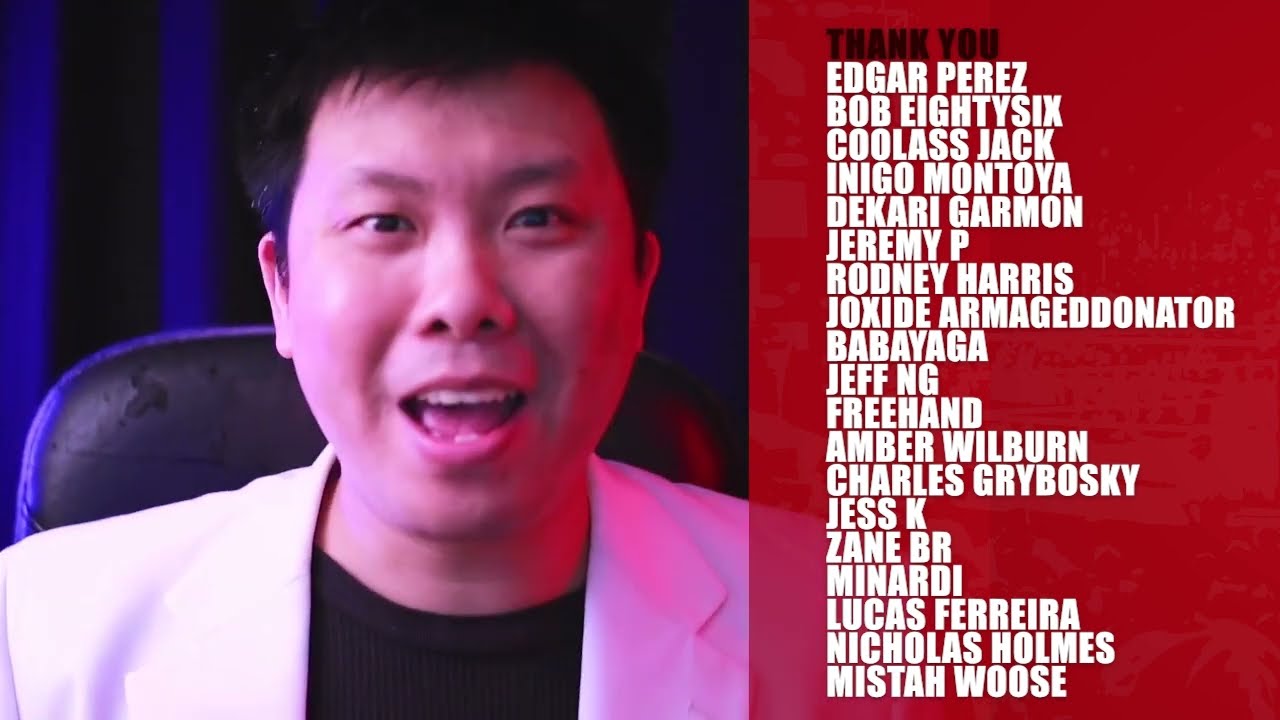The image features an Asian man with light skin, short black hair, and black eyes, sitting in a black leather or gaming chair. His attire consists of a white suit jacket over a black undershirt. He faces the camera with his mouth slightly open as if he's speaking. The background shows blue and black stripes with distinct blue and red lighting effects that cast a blue glow on the left side of his head and a red glow on the right side of his face. 

The left two-thirds of the image is occupied by the man, while the right third shows a transparent red box through which part of the man's shoulder is visible. This red section contains white text that lists names as a thank you: "Thank you, Edgar Perez, Bob 86, Cool Ass Jack, Indigo Montoya, Dakari Garman, Jeremy P, Rodney Harris, Jock C, Armageddonerder, Baba Yaga, Jeff NG, Freehand, Amber Wilburn, Charles Greiboski, Jess K, Zane B.R., Minardi, Lucas Ferreira, Nicholas Holmes, and Mr. Woos." The overall style resembles a CD cover, an album cover, or credits from a YouTube video.